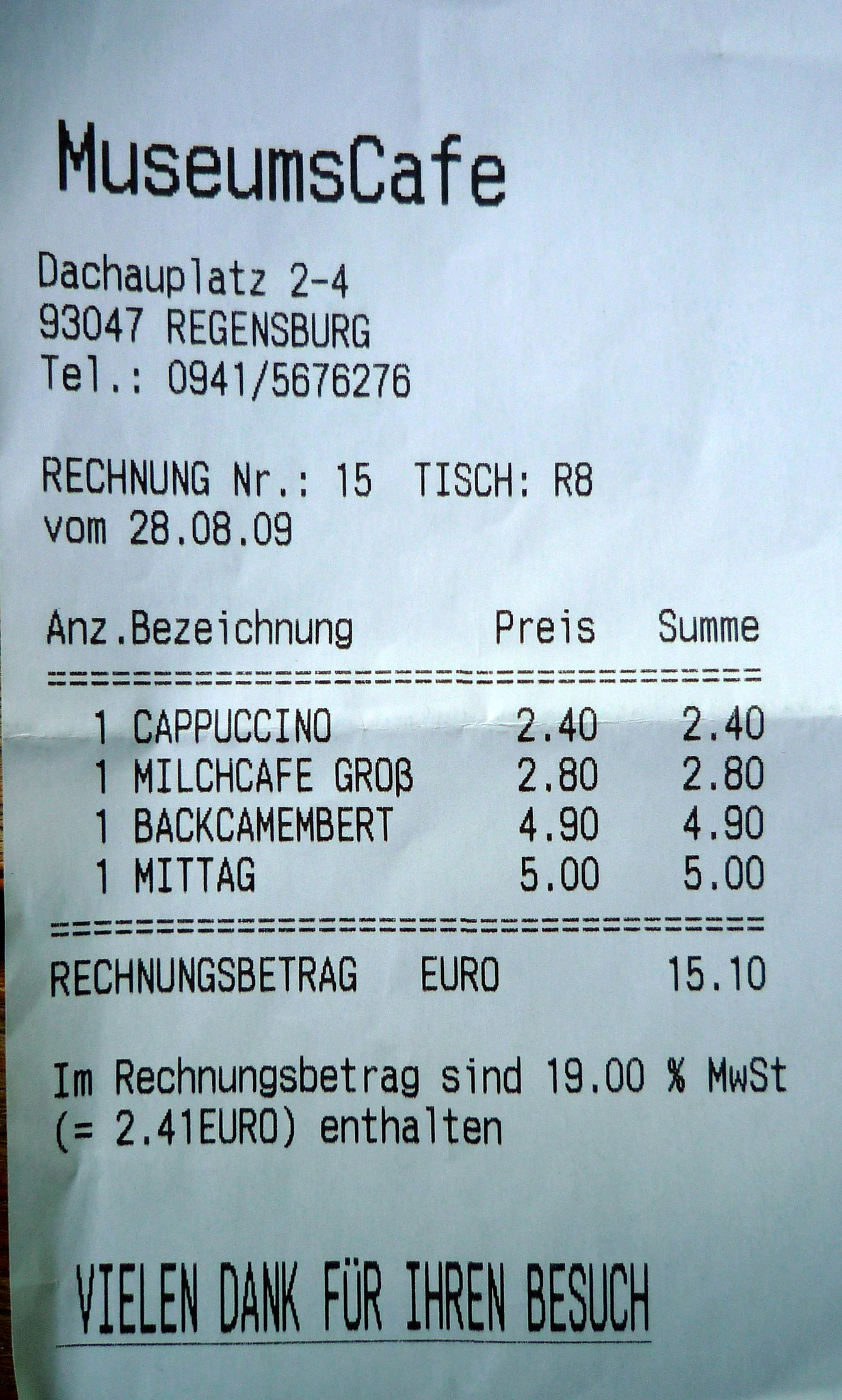This image features a detailed close-up of a receipt from a European establishment. The receipt occupies the entire frame, making it the sole focus of the picture. At the top, the receipt is identified as being from "Museums Café,” located at "Docco Plots 2-4, 93047 Regensburg." The contact telephone number for the café is listed as "0941 5676276." 

Key details on the receipt include:
- "Rich and node number 15"
- "Tish are 8" 
- "Vol 28/08/09" (likely a date)

Items purchased:
1. Cappuccino - €2.40
2. Milk Coffee (Milchkaffee) - €2.80
3. Cheese roll (Back Camembert) - €4.90
4. Lunchtime special (Mittagessen) - €5.00

The total amount for the purchase comes to €15.10.